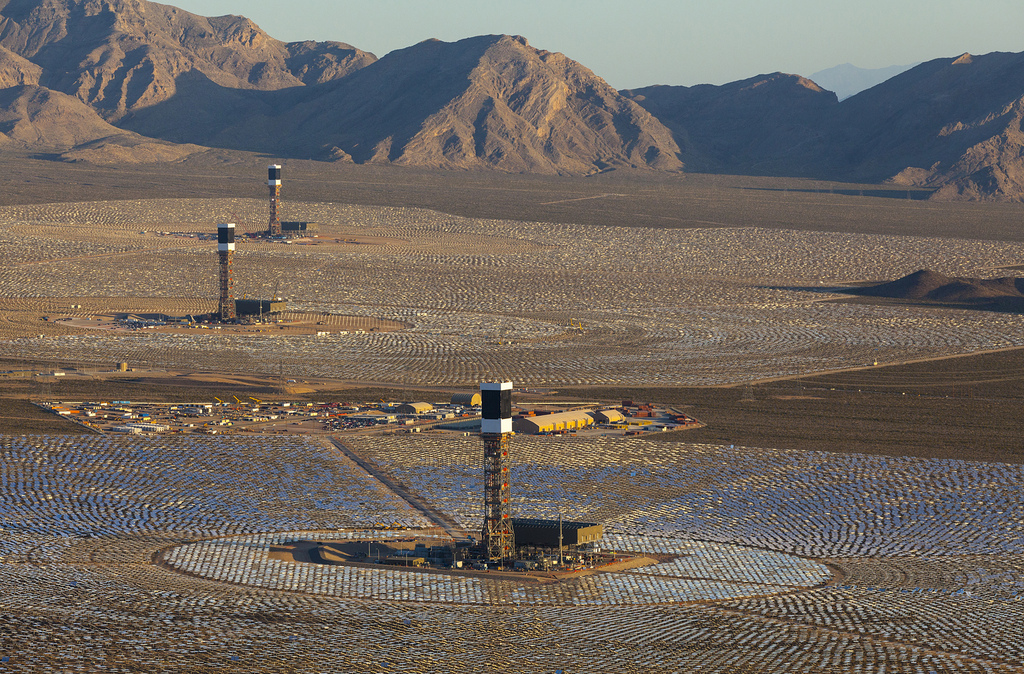This image, taken from a drone, captures an expansive and arid landscape in the Mojave Desert, featuring the Ivanpah Solar Electric Generating System. The terrain is dry, without any trees, and is dominated by three tall, slender, four-sided metal towers that have dark brown bodies with a vertical black section capped with white at the top and bottom. These towers overlook a sprawling field of solar collecting devices arranged in various rows. The central tower is particularly notable, as it is adorned with numerous red dots. Surrounding the middle tower are white industrial buildings, warehouses, cars, and conveyor belt machinery. In the background, the hazy light green sky contrasts with the desert hills and mountain ranges, contributing to the stark, arid atmosphere of the scene.